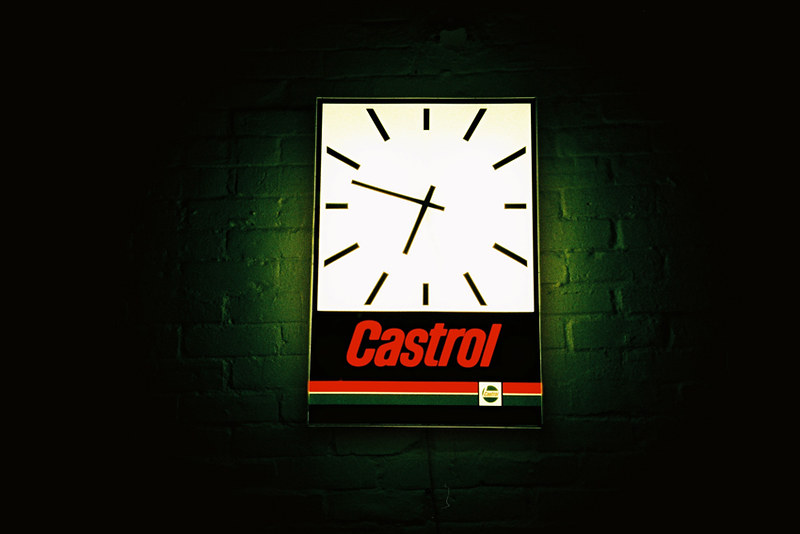The image showcases a white, vertical rectangular wall clock, brightly lit with a whitish halo that highlights the green brick wall behind it. The clock face lacks numbers, instead featuring golden lines to indicate the hours, and is adorned with gold and black minute and hour hands. Beneath the clock face, within a black rectangle, is the word "Castrol" in bold red letters. A series of stripes - red, thin white, and green - lines the bottom of this section, which also features the Castrol logo in a square with a white center. The edges of the clock are black, and the illumination from the clock casts an eerie greenish glow on the surrounding brick wall, which fades into darkness at the edges. The only text present in the image is "Castrol" along with the brand's logo.